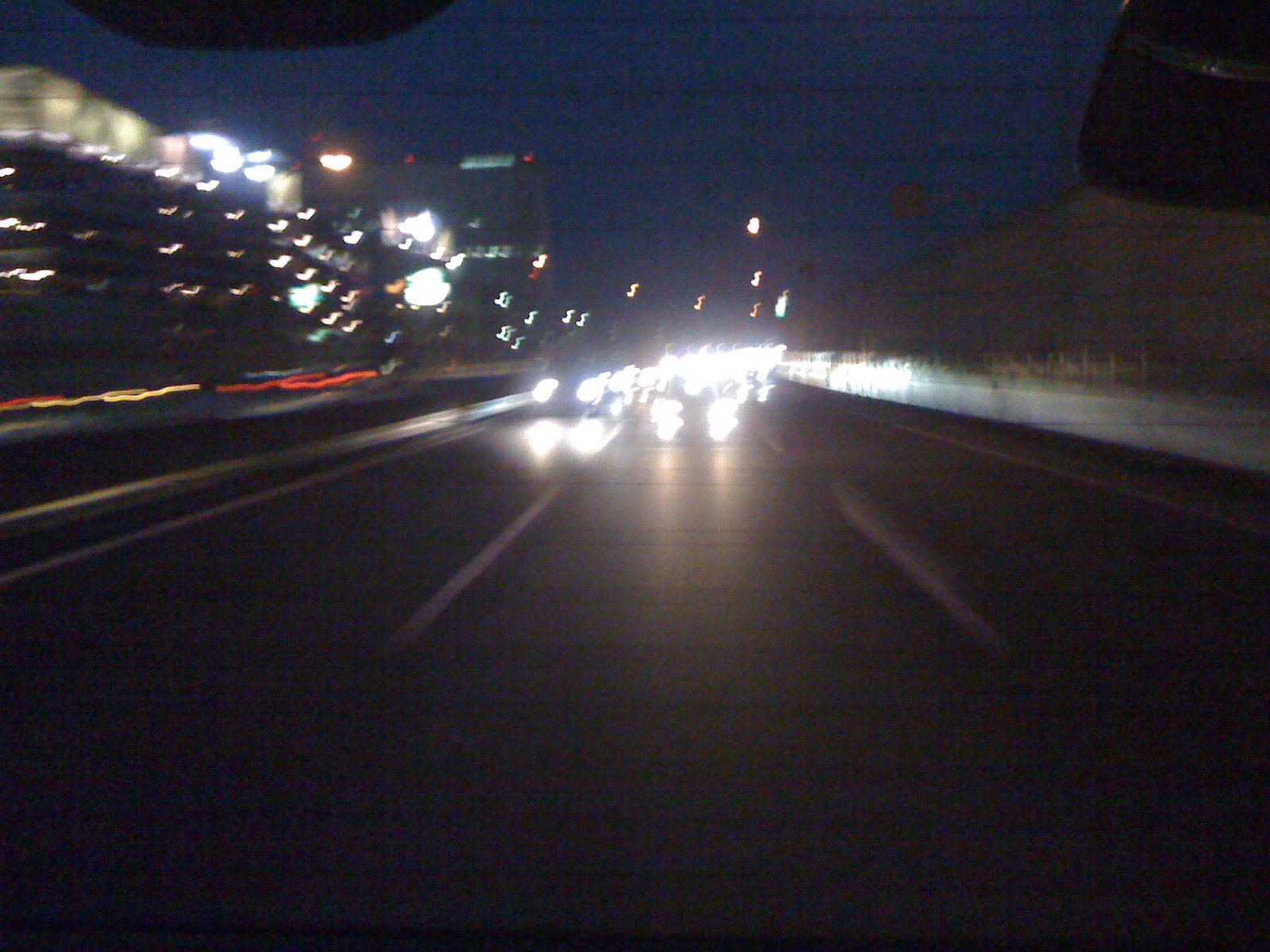A blurred nighttime photo captures the view from the rear of a moving car. The image is dominated by streaks of light from the headlights of oncoming traffic, which create artistic, music note-like patterns due to the camera's movement and limited exposure in low light. On the left, a stream of cars drives in the opposite direction, their lights adding to the visual cacophony. Amid the light trails, the outlines of tall buildings with illuminated windows stand faintly visible against the dark sky, while a wall spans the right side of the frame, grounding the scene in the urban environment.